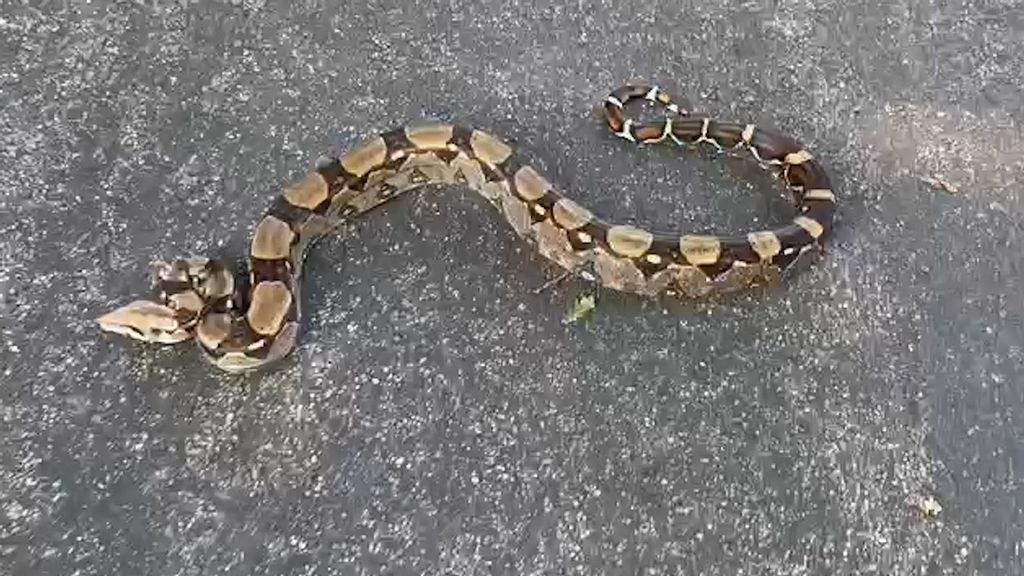This is an image of a large snake, which appears to be a rattlesnake, captured on a dark gray asphalt road, possibly a concrete street. The photo is taken from a top-down view, showcasing the snake coiling in a quasi-S pattern from left to right, with its pointed head on the left and its tail on the right amidst twigs, leaves, and rocks scattered around. The snake exhibits a distinctive checkered pattern, with greenish-brown segments interspersed with darker brown stripes. The lighter tan circles along its back become darker towards the tail, which ends with a segment containing yellow markings. Additionally, the underbody of the snake is light tan, contrasting against the black-topped road.